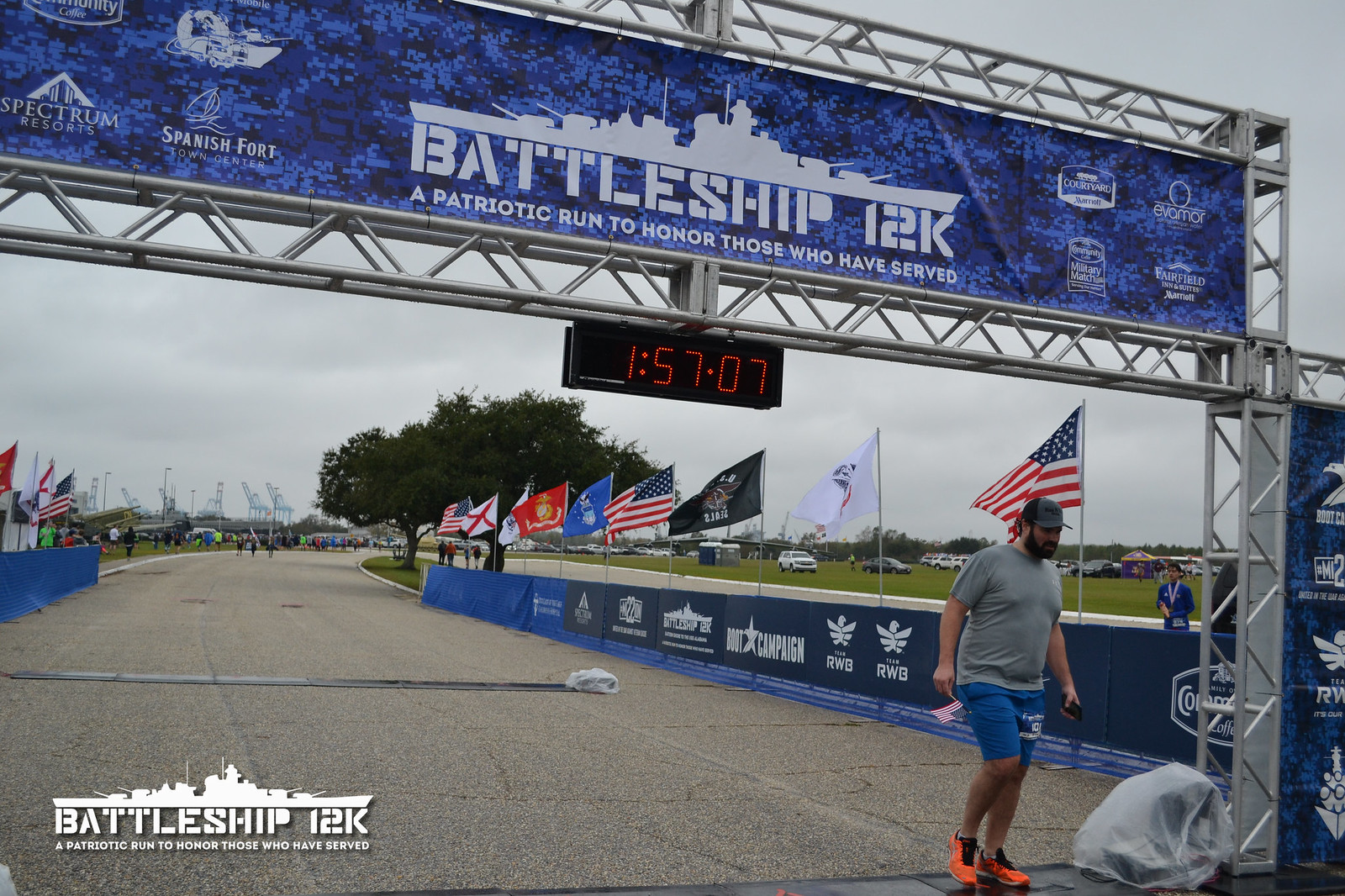The image depicts the finish line of the Battleship 12K, a patriotic run to honor those who have served. Dominating the scene is a blue banner supported by a metal structure, emblazoned with the event's name, "Battleship 12K," in white lettering along with the tagline, "a patriotic run to honor those who have served." Below the banner hangs a digital clock displaying the time 1:57:07 in red digits. Flanking the scene are various sponsors, including Spanish Fort Town Center, Spectrum Resorts, Fairfield Inn and Suites Marriott, Military Match, Courtyard Marriott, and Evamore.

In the foreground is a white male with a beard and mustache completing the race. He is clad in a gray short-sleeve t-shirt, blue shorts, a gray and black baseball cap, and bright orange trainers. The pathway is lined with flags from different countries, alongside American, U.S. Navy, and U.S. military flags. Spectators are seen behind barriers, observing the event, while additional runners approach the finish line. The sky is overcast but illuminated by daylight, and a grassy lot filled with parked cars occupies the background, adding to the sense of a large, communal event. An industrial area is vaguely visible in the distance.